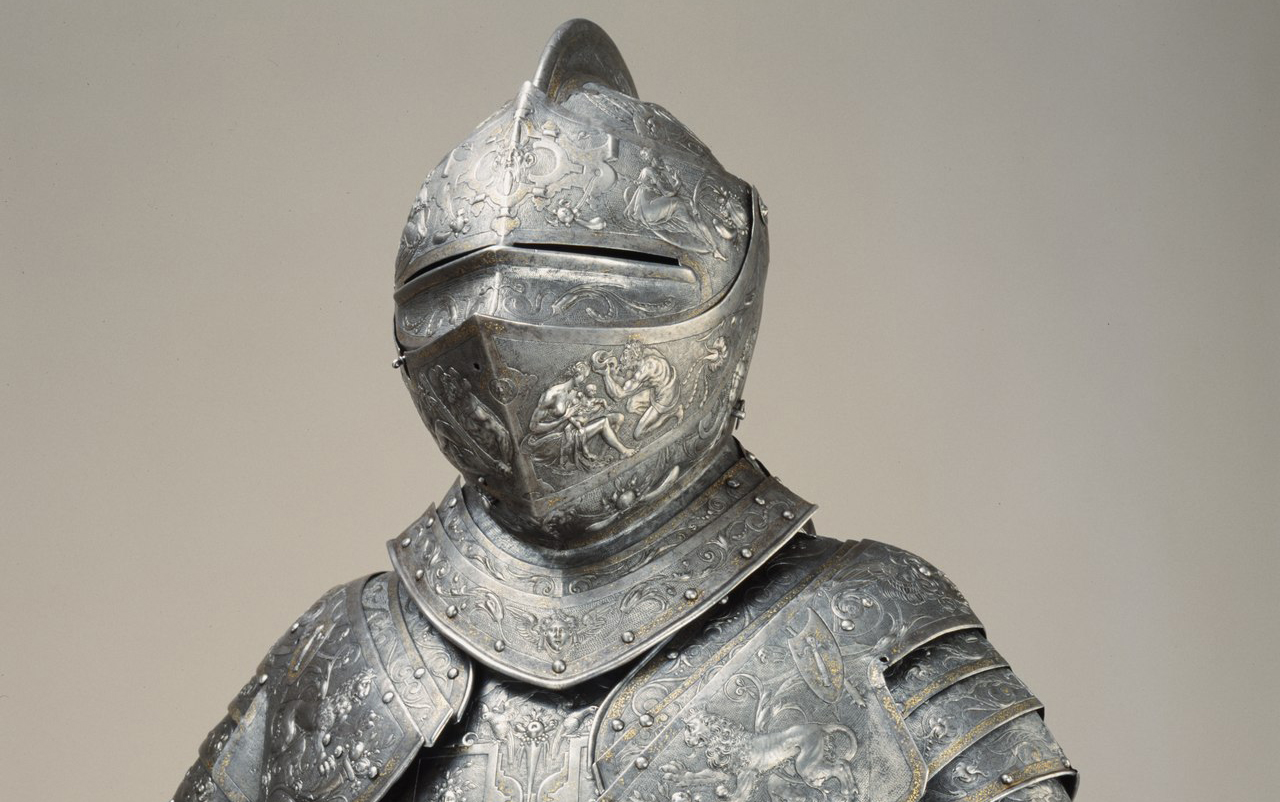The image depicts an intricate suit of medieval armor, primarily made of strong, silver-colored metal with elaborate carvings and golden detailing. The armor features heavy embroidery across the steel surface, with gold accents highlighting these areas. The visible sections include the helmet, chest plate, and pauldrons. The helmet incorporates dual eye slits, each separated at the center, and a distinctive disc in the middle. The chest and shoulder guards are adorned with various intricate illustrations, including images of angels with trumpets, lions, a man's face on the armor, and a woman's face located at the junction of the chest plate and neck piece. Figures of a man holding a snake, a skinny man with prominent ribs, and a woman with a child are also part of the ornate carvings. The armor, likely displayed in a museum with a tan background, appears to cover the knight fully from the chest up, ensuring comprehensive protection while also allowing for arm movement due to the design of the shoulder guards.